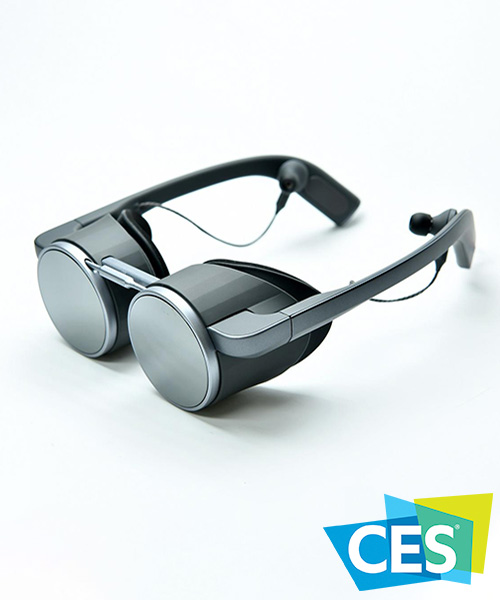This photograph showcases an innovative futuristic device that resembles a pair of eyeglasses but is identified as a virtual reality headset. Dominating the image, the headset features cylindrical lenses where each lens is perfectly circular. The eye area, crafted from a dark, thick metal, juts out significantly from the frames, allowing space for intricate electronics within. The arms of the headset, which are thick and robust, extend back over the ears with wires running down each, ending in earbuds designed to fit into your ears. The image background is a clean white that contrasts vividly with the device's dark metal. Notably, the bottom of the photograph displays the CES logo in white text, indicating its association with the renowned Consumer Electronics Show, set against a blue and green backdrop. The composition and elements strongly emphasize it's a cutting-edge virtual reality device.